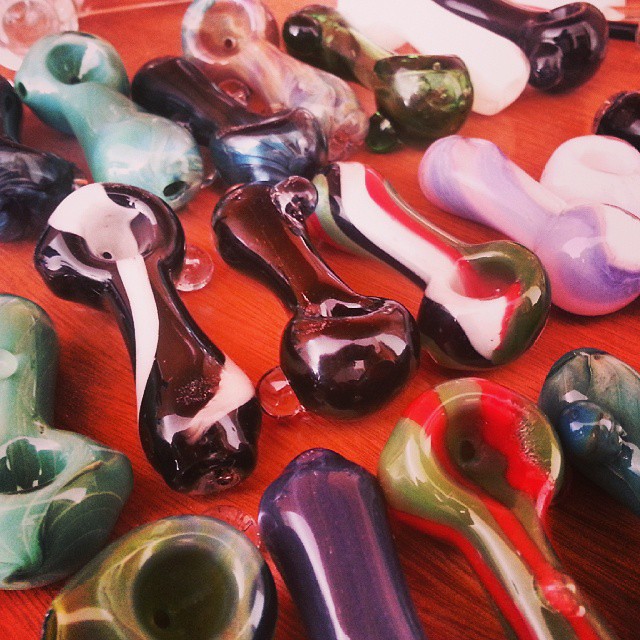The image showcases an up-close display of 19 hand-blown glass pipes, typically used for smoking various substances, arranged diagonally in three distinct rows on a reddish-brown wooden surface. Each pipe bears intricate designs featuring lines, striations, and bumps, with colors ranging from black, white, green, and gold to light pink, purple, and red. The pipes, often shaped like small spoons with rounded tops and a bowl with a central hole, are illuminated well, suggesting they might be placed in a display case. A few of the pipes in the middle row have beads of water on them, adding to their vibrant, pearlescent appearance. The setting is clearly indoors, focused on highlighting the detailed craftsmanship and vivid colors of these glass pieces.